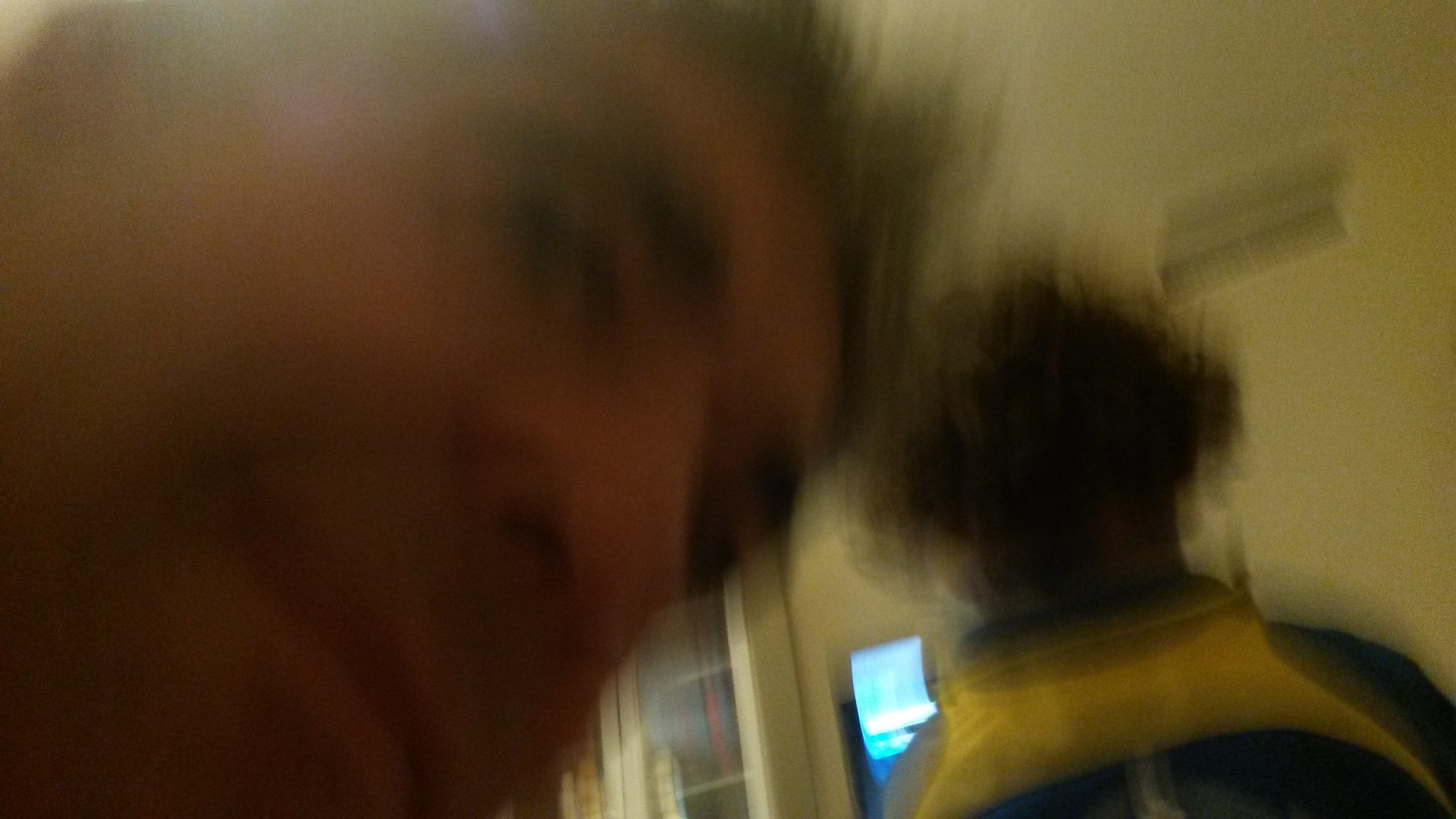This image depicts a highly blurred scene featuring two men. The prominent figure, an older man with short brown hair and bushy eyebrows, occupies most of the left side of the frame. His face appears large due to his proximity to the camera, and he is angled towards the right while flashing a grin at the lens. In the background, on the right side of the photograph, another man with very curly hair can be seen sitting behind a desk, engaged in playing a game. He is dressed in a blue jacket with yellow accents, and the faint glow from a computer screen illuminates the left side of the scene. The setting seems to be indoors, with a white wall backdrop and two large rectangular vents visible near the top of the image. Overall, the photograph captures a moment between two individuals, though the severe blurriness of the image obscures finer details.